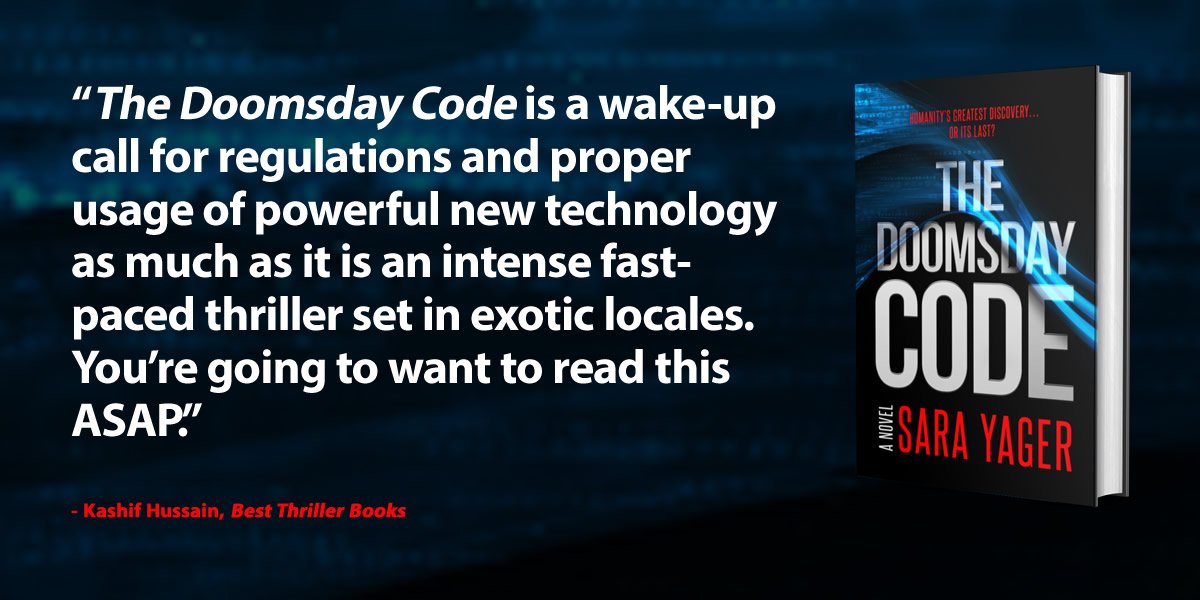This image is an advertisement for the book "The Doomsday Code," a novel by Sarah Yeager. The right side of the horizontal rectangle prominently features the book cover, which includes blue, black, and red elements, possibly depicting smoke or waves of water. A tagline in red is situated at the top of the book cover. The left two-thirds of the image contain a testimonial in white text from Kashif Hussain of Best Thriller Books, declaring, "The Doomsday Code is a wake-up call for regulations and proper usage of powerful new technology, as much as it is an intense, fast-paced thriller set in exotic locales. You're going to want to read this ASAP." This text, attributed in red to Kashif Hussain, contrasts against a deep blue, subtly wavy background.